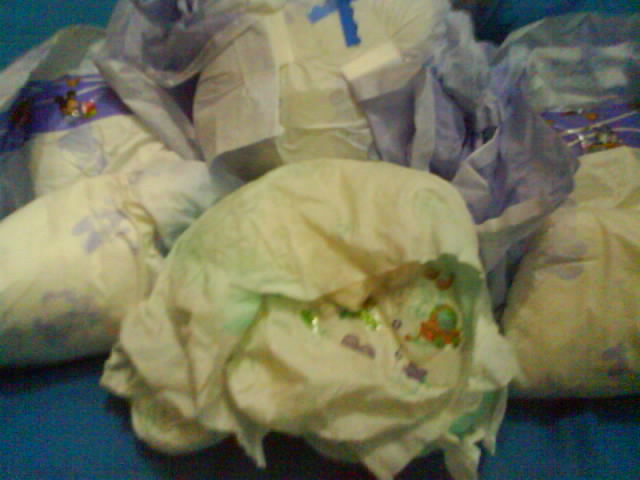The photograph depicts what appears to be a collection of items wrapped in colorful paper, likely disposable diapers, potentially mistaken for cheeses or tissue paper. The items are predominantly enclosed in yellow paper with green accents, although some are wrapped in lavender paper as well. One of the yellow wrappings is open, revealing diapers inside, adorned with small cartoon figures and some plasticky material. The diapers, appearing folded and possibly used, are gathered in a bunch on what looks like a royal blue surface, possibly a counter or table. Despite the photo being slightly out of focus, it’s clear that there are about five or six items. The most prominent item at the front displays a label with images in red, purple, and green hues alongside a large "L" at the top. The overall scene seems like a random assortment of bunched-up, potentially used disposable diapers, wrapped in varied tissue or wrapping paper, situated on a blue background.